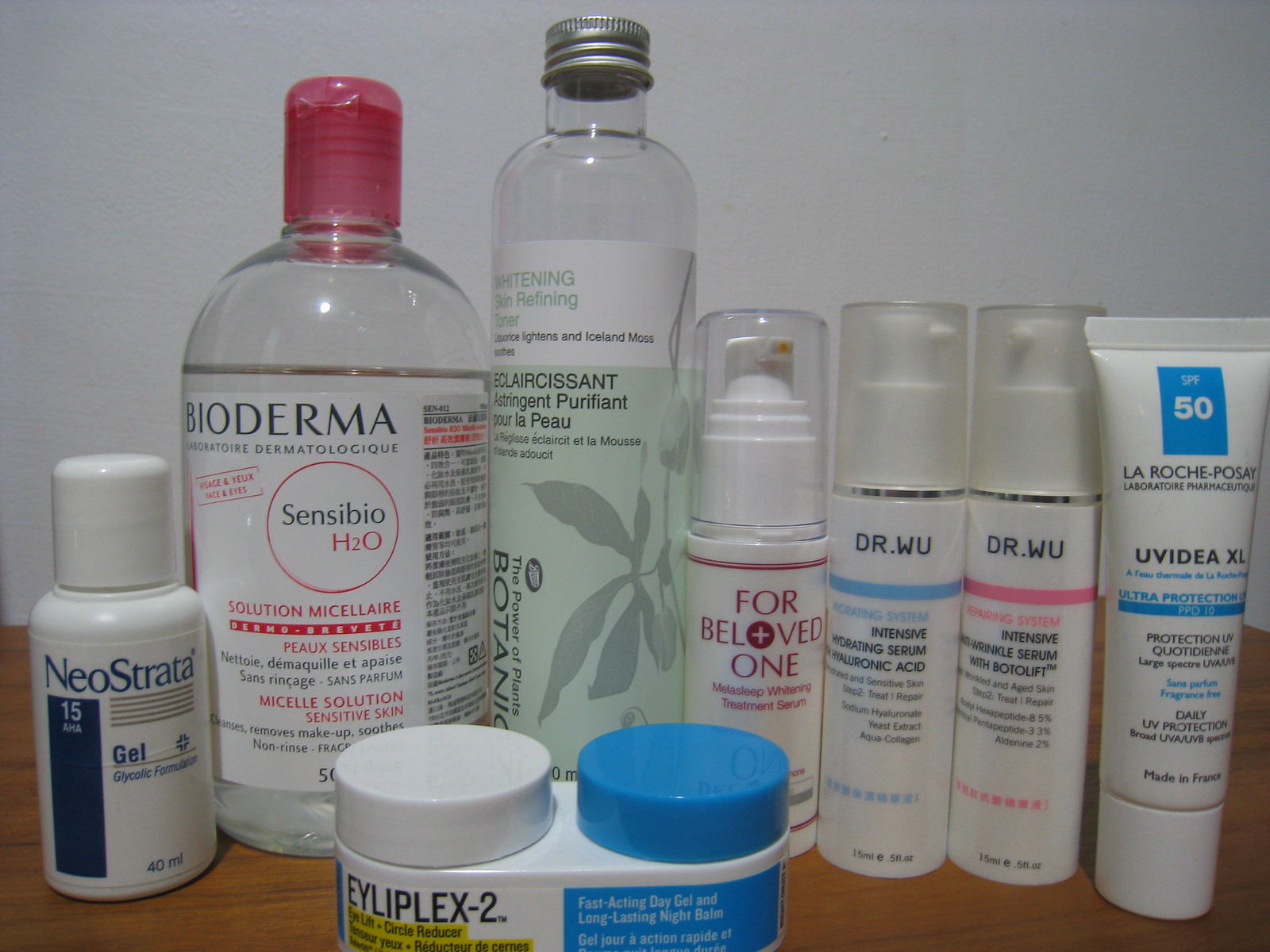A neatly arranged display of skincare and body products sits on a wood-grain surface, which appears to be a shelf or table, against a simple white wall background. The photograph, which is wider than it is tall, showcases seven tubes of skincare products aligned in a row. From left to right, the brands and products visible are: 

1. NeoStrata
2. Bioderma
3. Botanic for Beloved One
4. Dr. Wu (three different products)

In the foreground at the bottom of the image, there is an additional product labeled "EYIPLEX-2," which features a white cap and a blue cap, likely a container for a fast-acting day gel and a long-lasting night balm. The tubes' labels vary in color from white to clear, suggesting a cohesive, clean aesthetic. This meticulously organized display of skincare items awaits use, promising a thorough skincare routine.